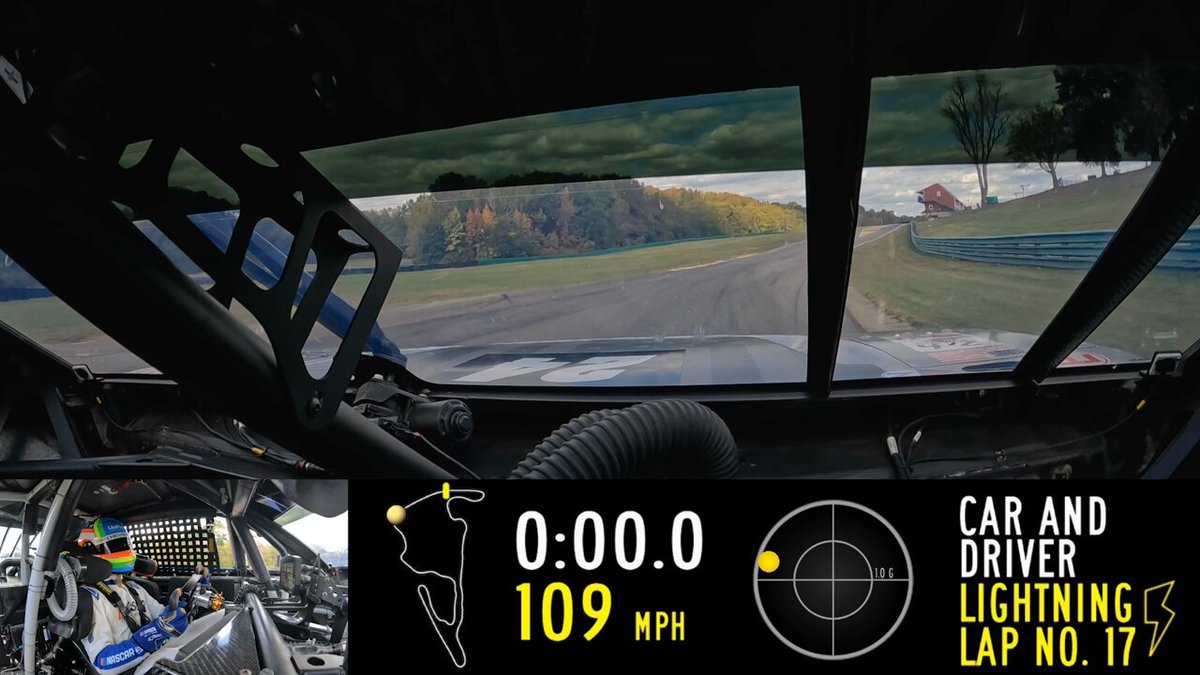This image depicts a vivid, detailed point-of-view scene from inside a race car, showing the road ahead from the driver's perspective. The foreground showcases the car's dashboard filled with various information, including a black circle with a small yellow center, displaying "0:00.00" in white and a speed of "109 miles per hour" in yellow. Prominently displayed is the phrase "Car and Driver Lightning Lap Number 17." The driver, clad in full racing gear, including a helmet and safety equipment, grips the steering wheel within the protective framework of the car's cage. Outside the car, the scenery features a single country road bordered by green fields, trees, a low blue fence on the right, and a small hill. In the farther distance, a red structure that resembles either a barn or a pit stop is visible, adding to the rural and dynamic ambiance of the scene. The entire image has a subtly painted quality, enhancing its dynamic and immersive feel.